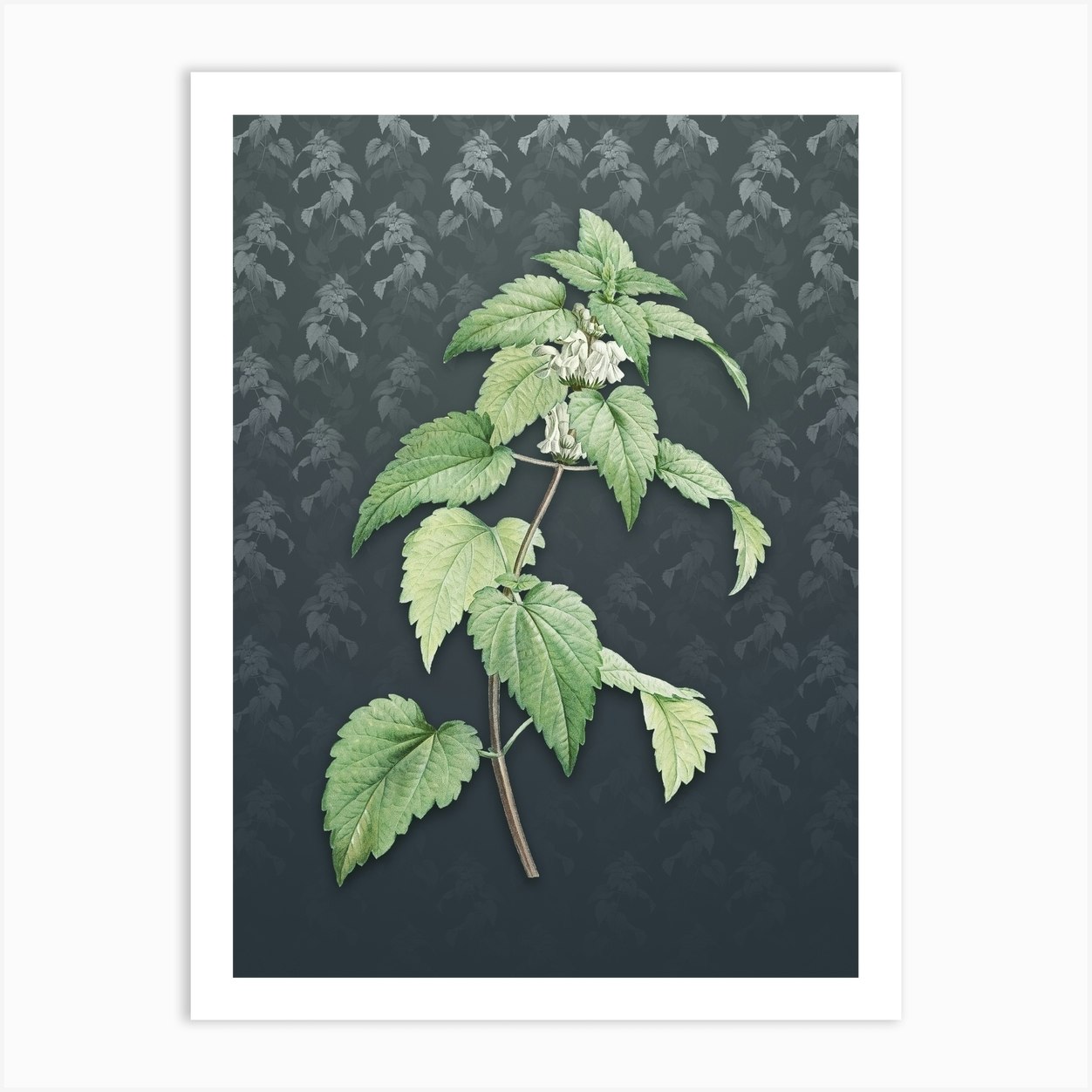The image showcases a detailed and vivid painting of a green nettle plant, prominently positioned against a dark gray, nearly black background. The central plant has jagged, heart-shaped leaves, rendered in multiple shades of green to highlight the intricacies of its foliage. Towards the top, delicate white, bell-like flowers dangle from the stems, enhancing the plant's lifelike quality. The background intriguingly features faded silhouettes of additional nettle plants, creating a sense of depth and texture. This digital artwork appears meticulously cropped onto a crisp white page, giving the impression of a white canvas bordered by a white wall. The overall composition is harmonious, with the bright, realistic colors of the central plant contrasting effectively against the subtle, shadowy hues of the background foliage.